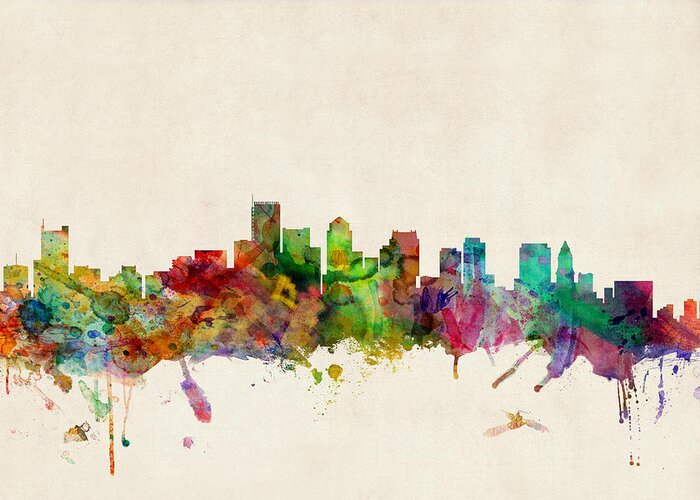The image showcases an abstract watercolor painting set against a tan, possibly off-white or eggshell white background. It features a multicolored depiction of high-rise buildings, reminiscent of a city skyline, possibly New York City. The vibrant array of colors includes blue, green, red, yellow, orange, purple, light blue, pink, and black, creating a rainbow-like palette that drips and blends in places, adding to its abstract nature. The painting occupies the lower portion of the image, spanning from one side to the other but not centered. There is no text or framing, allowing the colorful, messy rendition of the urban landscape to stand out dynamically against the neutral background.